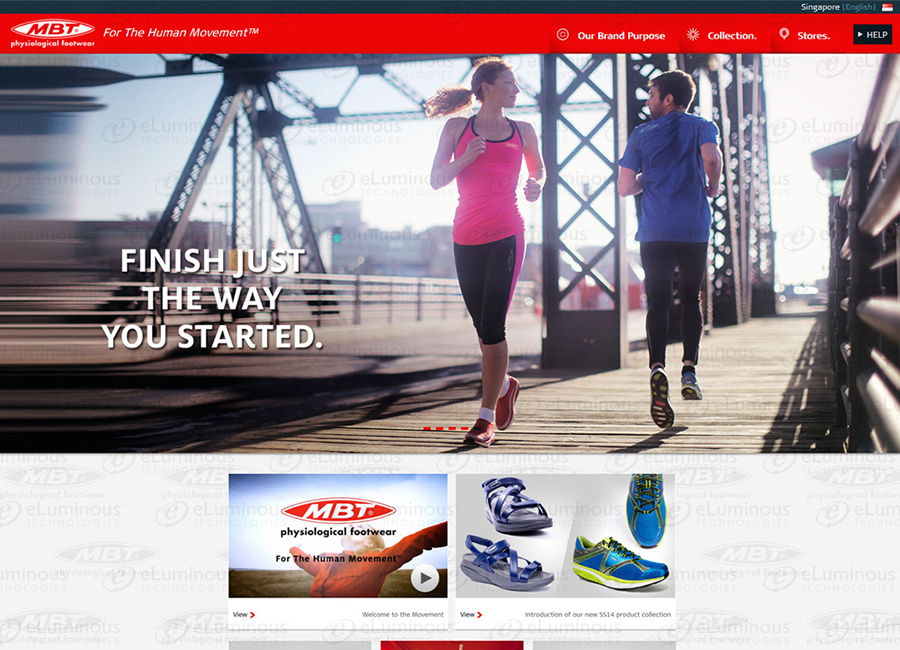This is a detailed description of a website screenshot designed for promoting running shoes. The top bar features a black line, followed by a red banner with white text that reads, "For the Human Movement, Our Brand Purpose, Collection, Stores, Help." Just beneath this, there's an image capturing two runners passing each other on a wooden bridge, accompanied by the motivational message, "Finish just the way you started."

Further down, the background transforms into a transparent wallpaper featuring the logo "MBT, Psychological Footwear for the Human Movement." Centred on this section is a play button labeled "View," inviting users to "Welcome to the Movement."

Adjacent to this, there are images of sandals and running shoes, each paired with a red arrow guiding the viewer to explore these product collections further.

Continuing down the page, there are three distinct sections: a gray box, a blue and red box, and another gray box, adding structured elements to the website's layout.